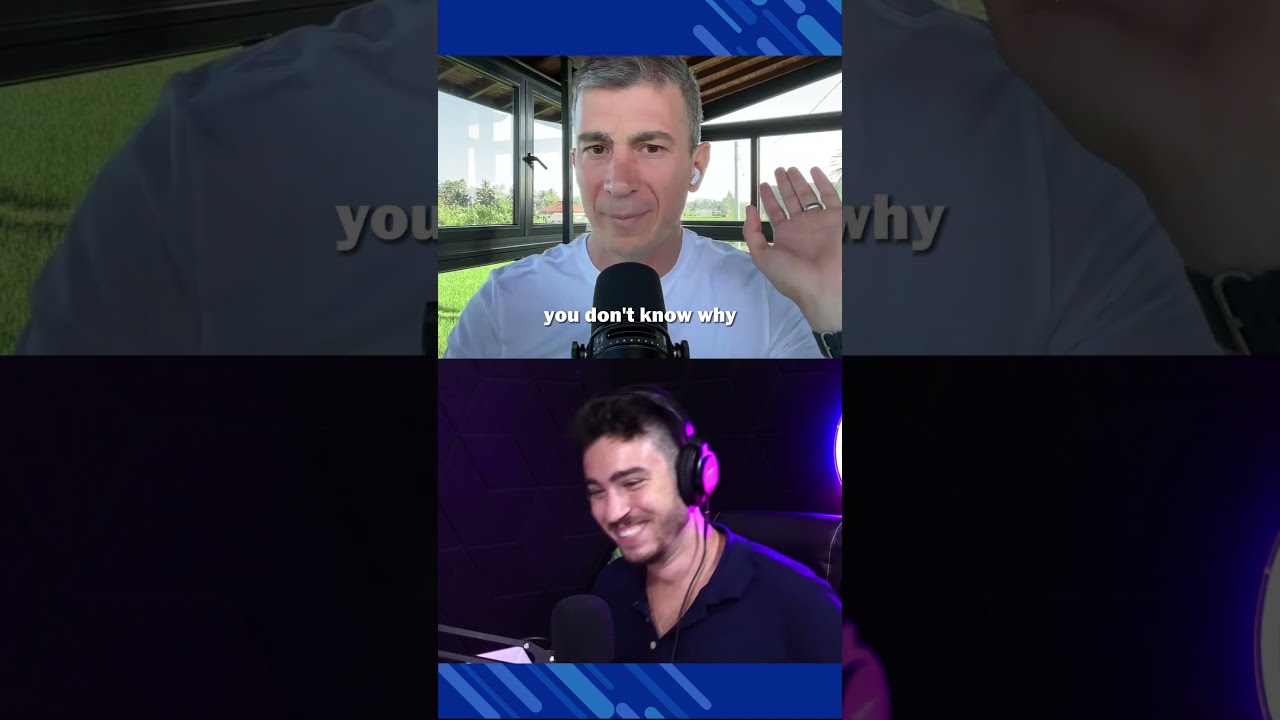The central image showcases two vertically stacked photographs of Caucasian men, set against a dimly lit background. The upper picture features an older man with thin gray hair, thick brownish eyebrows, and apple earbuds. He's dressed in a white t-shirt, has a ring on his ring finger, and is waving with his right hand. Positioned in front of him is a black microphone, and subtitled in white text just below his chin are the words, "you don't know why." The lower photograph shows a younger man with short black hair and slight facial hair, wearing black headphones that reflect a pinkish hue from the ambient lights. He dons a navy blue polo shirt and has a black microphone in front of him. Both men appear to be participating in a streaming interview, with their individual images highlighted in the central rectangular frame while fragmented repetitions of their images form the dimly lit dark navy blue and black background.